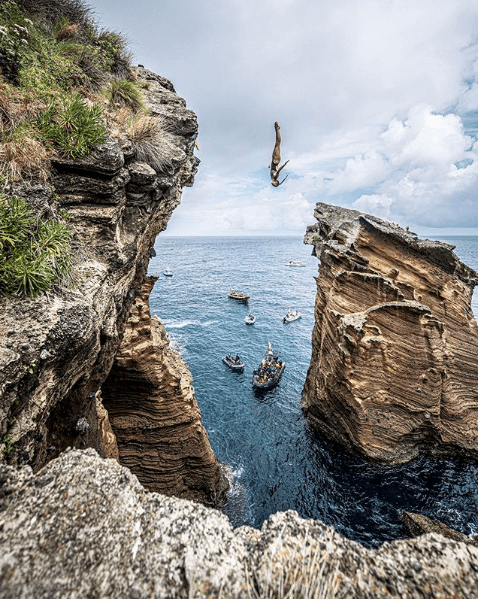The photograph captures a dramatic scene of a cliff diver in mid-air, head down, plummeting towards the blue ocean below. The diver is positioned between two rugged cliffs - one occupying the left third of the frame and adorned with sparse grasses and shrubs, while the other, a smaller island cliff, rises from the water on the right. The rough texture of the cliffs contrasts with the expanse of ocean beneath, which is dotted with several ships of varying sizes. The scene is viewed from another cliff edge, offering a comprehensive lookout. The overcast sky is thick with clouds, though occasional patches of blue are visible, adding to the moody atmosphere of the image.